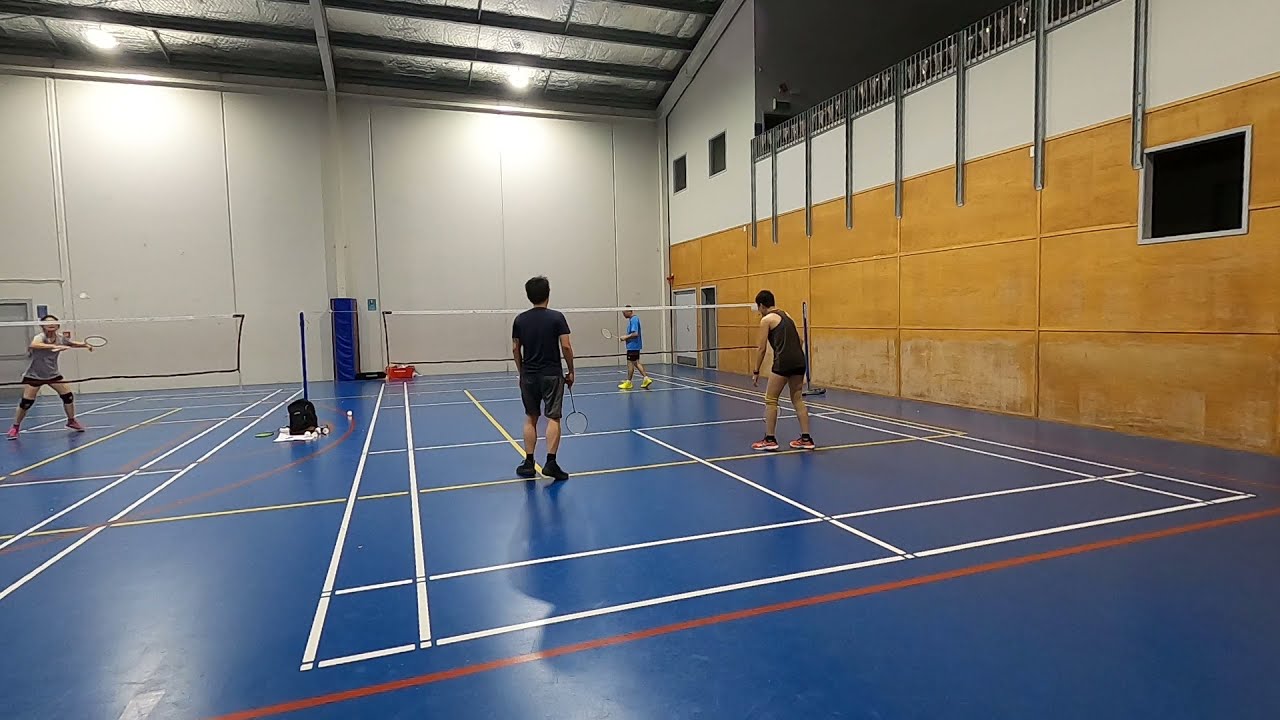The photograph showcases an indoor badminton game set in a spacious, high-ceilinged gymnasium with a partially unfinished ceiling, where lights hang down to illuminate the scene. The floor is a deep blue, interlaced with white, red, and yellow lines designating the boundaries of the courts. The image prominently features a doubles match in the center, where all players appear to be men dressed in casual athletic wear. Notably, one player sports a black muscle shirt, and another stands out with yellow sneakers and a blue t-shirt. On the left side of the image, a second court is visible with a player poised to hit an incoming birdie. The gym's walls have a distinct design: the upper portions are white, while the lower sections are a tan brown hue. Athletic bags lie scattered outside the court lines, likely containing extra gear or shuttlecocks.